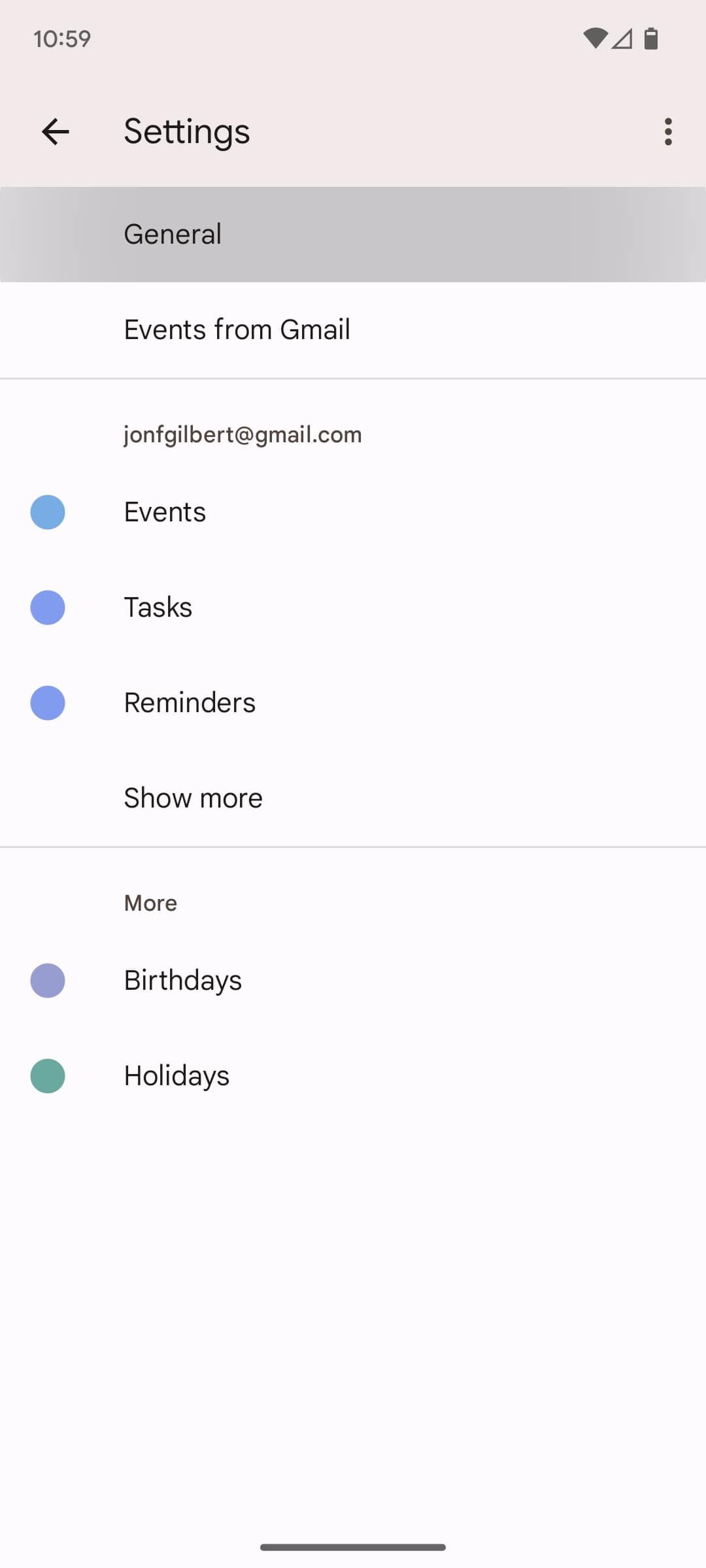The image is a screenshot from a cell phone's display. At the very top, there's a light gray header. In the upper left corner, in dark gray text, the time reads "10:59." In the upper right corner, there are a black Wi-Fi icon indicating a connection and a nearly full battery icon. Just below the header, large black text reads "Settings" with an arrow pointing to the left, indicating a back navigation option.

Beneath the "Settings" label, there is a darker gray banner with the word "General" written on it. Against a white background below this banner, there is the text "Events from Gmail" followed by a narrow horizontal gray line. Under this line, it shows "John F. Gilbert" with the email address "john.f.gilbert@gmail.com."

Moving further down, there are options listed from top to bottom: "Events," "Tasks," and "Reminders," each accompanied by a blue circle to the left, except "Reminders," which has a blue circle to the right. Below these options, "Show More" is written in black text followed by another thin horizontal gray line.